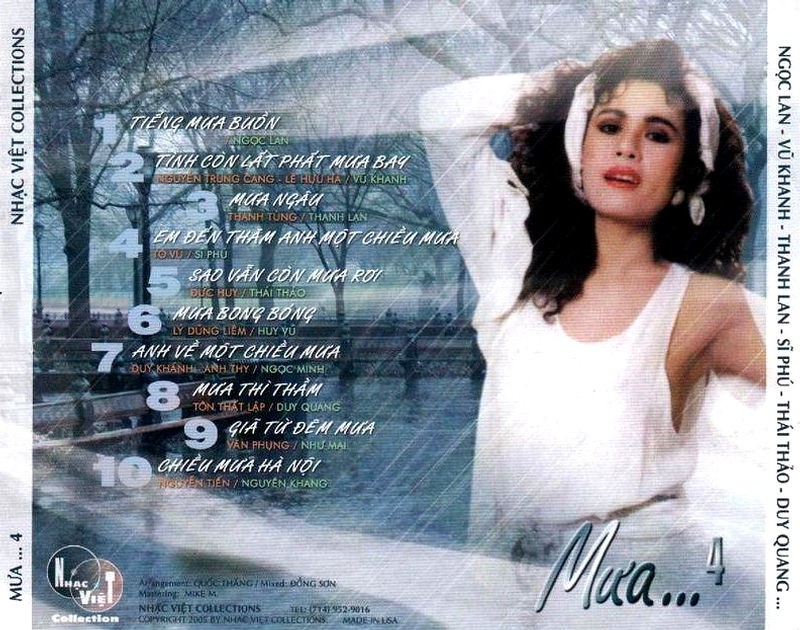An apparent CD cover showcases a Caucasian female on the right, posed with her right hand behind her head and her left arm extending off the image. She dons a white tank top, a white headband, and a white item draped over her shoulders. The woman has long, curly brown or black hair and is wearing full makeup, with her mouth slightly open and her head tilted back. Beneath her image, the text reads "MUA..." followed by the number 4.

The background presents an outdoor scene with dead trees and park benches on what appears to be a rainy day, with diagonal white lines suggesting rain. On the left side of the cover, there are numbered song titles listed from 1 to 10, written in white and followed by colored text, presumed to be in Vietnamese.

On the left and right borders, there is vertical text. The left border includes the phrase "N-H-A-C-V-I-T collections" at the top, and an interconnecting circle design with illegible letters in white text near the bottom left. The overall color scheme of the background is predominantly blue and gray, enhancing the moody and atmospheric feel of the image.